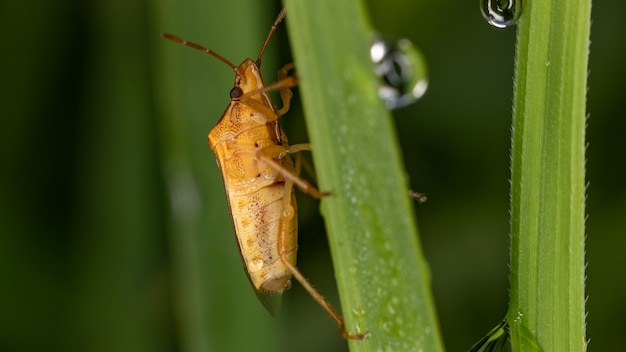This image is a highly detailed, close-up photograph of a bug climbing on a green plant stalk, which appears to be a blade of grass. The bug, possibly a cricket or stink bug, is predominantly orangish-tan in color with varying shades of brown. It has two long brown antennae and a single visible black eye. The bug’s head is a darker brown, transitioning to a lighter brown towards its tail, with the tip of the tail being a very dark brown. Its six legs cling tightly to the left side of the central plant stalk, which is in sharp focus.

The plant itself has fine hairs visible due to the high level of zoom. There are four plant stalks in the composition: two near the left, which are slightly out of focus and darker, and two on the right, which are more centered and in focus along with the bug. Each of these focused stalks has a large water droplet rolling down their sides. The background of the image, which is out of focus, shows more of the plant, adding depth to the photograph. Overall, the image captures not only the intricate details of the bug but also the vividness and texture of the plant and water droplets.